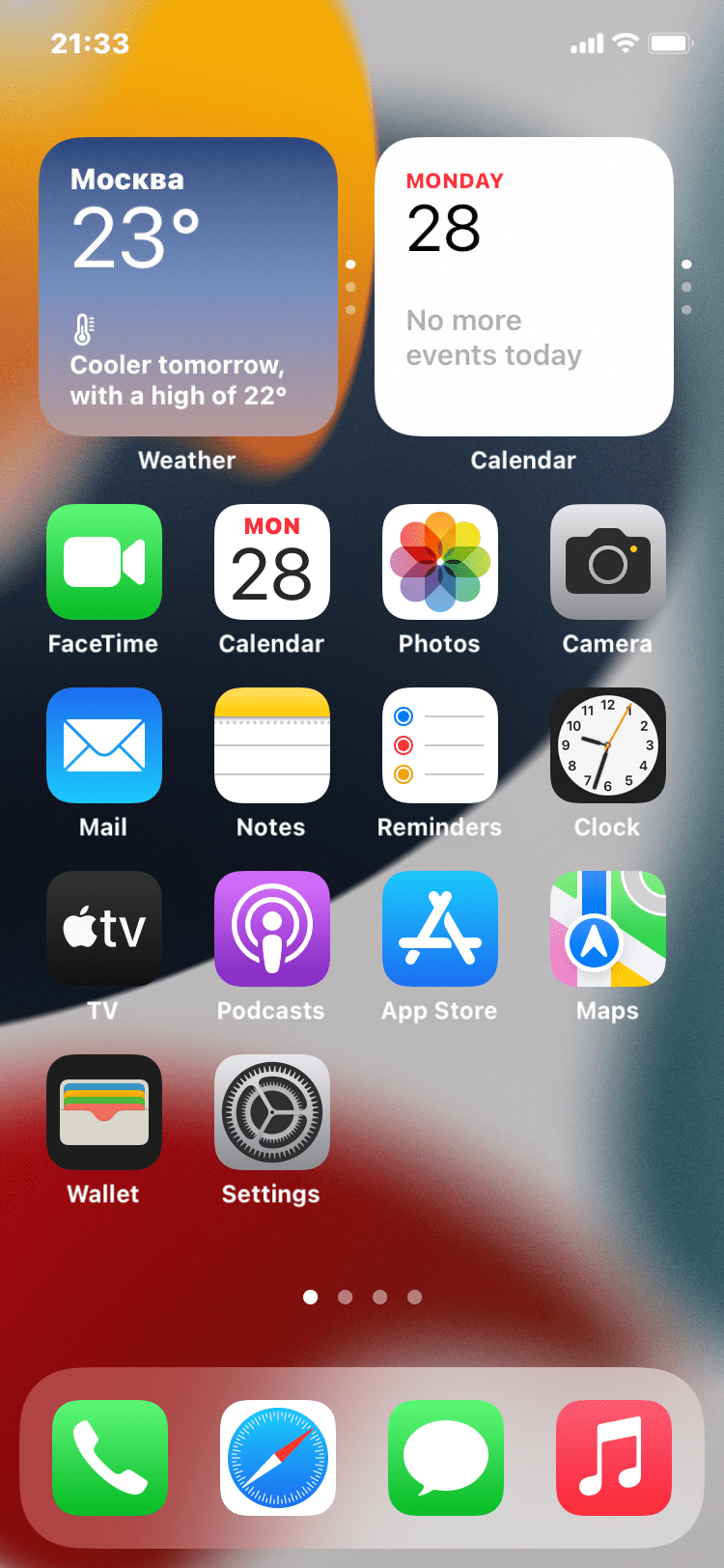This image is a detailed screenshot of an iPhone home screen, likely from an older model, possibly an iPhone 6 or 7. The background is a vibrant mix of colors including yellow, black, gray, white, and red at the bottom. The time displayed is 21:33, and the phone is connected to Wi-Fi with a full signal and battery.

At the top of the screen, there are two widgets: one showing the weather and the other displaying the calendar. The weather widget indicates the temperature in "МОСКВА" (Moscow in Cyrillic), with the temperature currently at 23 degrees Celsius and stating "Cooler tomorrow at a high of 22 degrees." Next to it, the calendar widget reads, "Monday 28th, no more events today."

The main screen is organized into four rows of app icons, with each row containing four apps, except for the last row which has only two. The apps are as follows:

- **First Row:** FaceTime, Calendar, Photos, Camera.
- **Second Row:** Mail, Notes, Reminders, Clock.
- **Third Row:** Apple TV, Podcasts, App Store, Maps.
- **Fourth Row:** Wallet, Settings.

Beneath these app icons, there are four dots indicating multiple home screen pages.

At the very bottom is the dock, containing four apps: Phone, a blue circle with a red and white clock (potentially the World Clock or an international time app), Messages, and Apple Music.